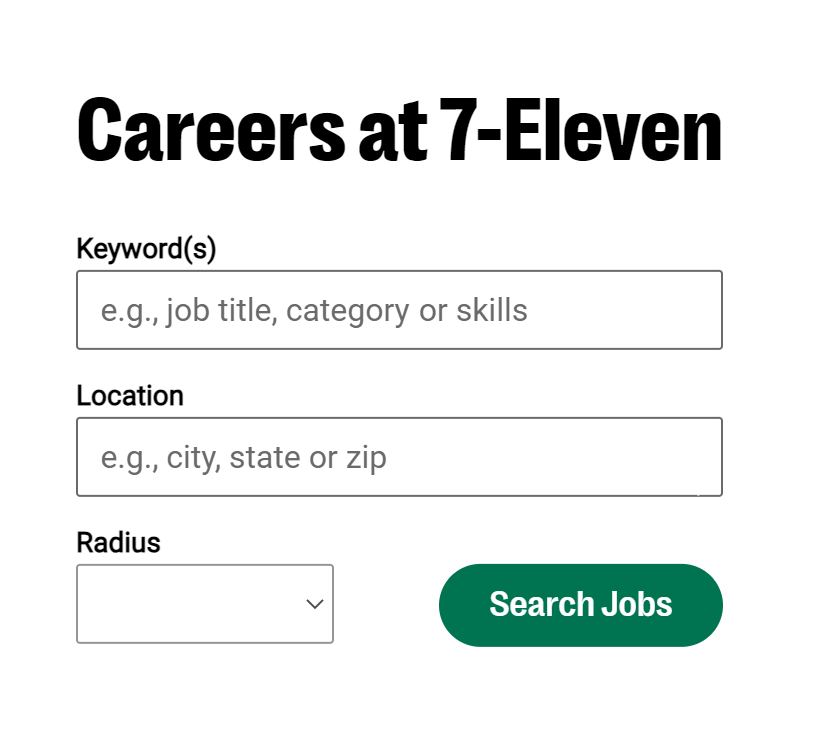The image features a minimalist layout against a plain white background, dominated by a job search interface for 7-Eleven. At the top, bold black text reads "Careers at 7-Eleven." Below, there's an input field labeled "Keyword(s)" that allows users to enter job titles, categories, or skills, accompanied by a white text box for input. Underneath, the form includes another input field labeled "Location" with an example placeholder text "e.g., city, state, or ZIP code" and a corresponding text box. Further down, a "Radius" selection field includes a dropdown icon on its right side for users to choose the search radius. To the right of this radius field is a long, oblong-shaped button in a teal dark green color, bearing the text "Search Jobs" in white. The rest of the interface is uncluttered, featuring significant empty space, which keeps the focus on the job search functionalities.